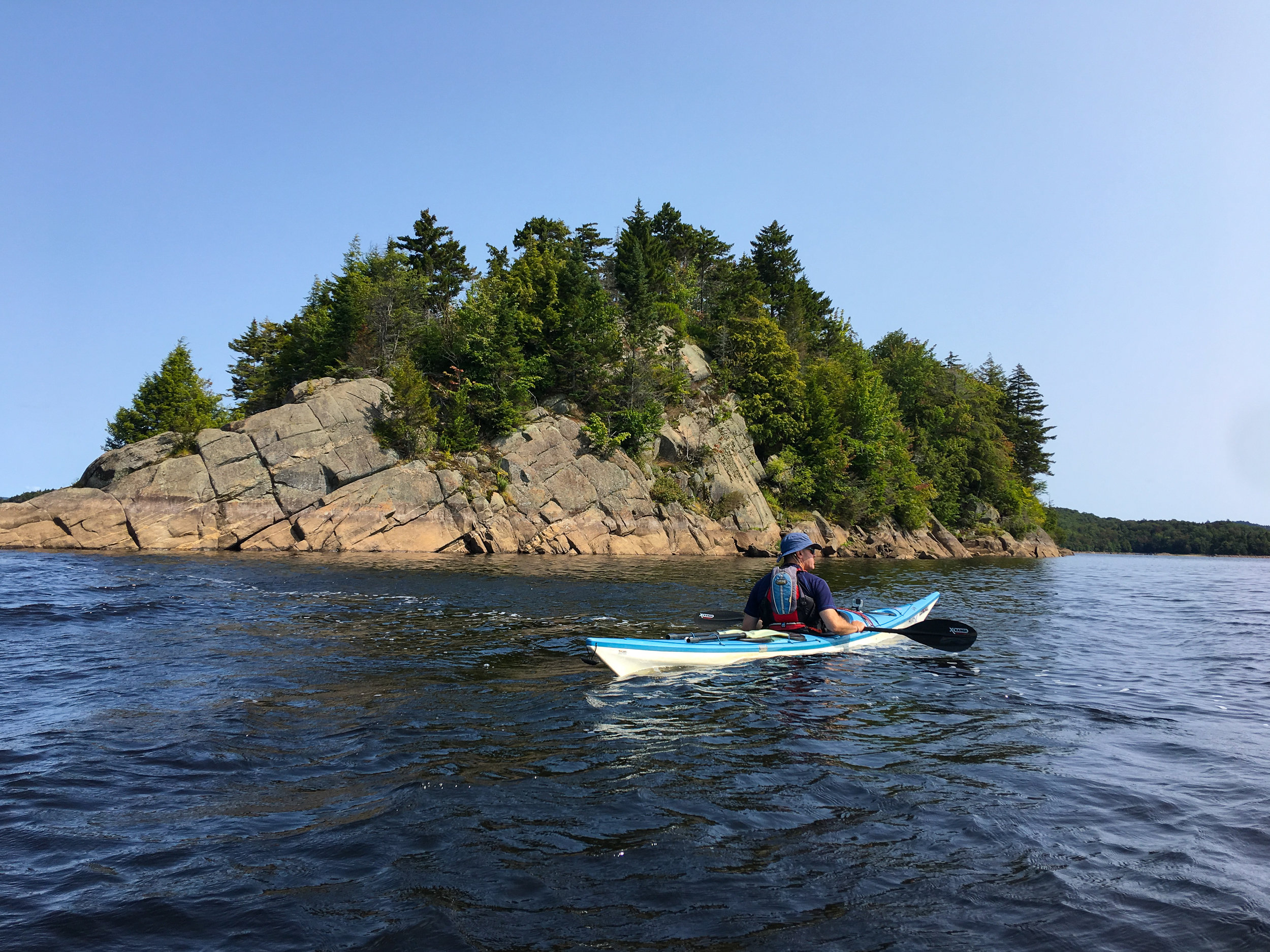A man is kayaking in a two-toned kayak, with the top in light blue and the underside in white. He wears a dark blue short-sleeved t-shirt, paired with a matching blue boat hat. Black sunglasses shield his eyes from the sun, and a black paddle rests horizontally across his lap. The water he navigates is a dark brown and slightly choppy, adding a sense of movement to the scene. In the background, rugged cliffs and large rocks stand tall, adorned with trees in varying shades of bright and dark green. The dense wooded area extends to the right, featuring a vibrant mix of light and dark-leaved trees. The man's gaze is directed towards the right side of the image, positioning him centrally both within the foreground and background.